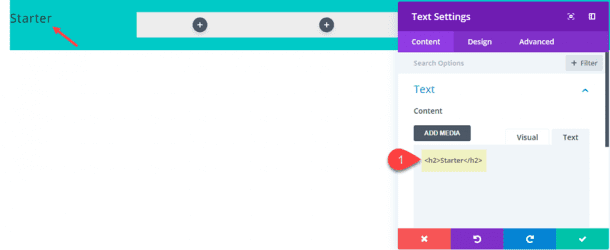The screenshot image captures a webpage with a predominantly white background and various labeling in aqua, purple, and light blue hues. At the top of the image, an aqua bar extends horizontally, interrupted by a white strip in the center with two plus signs inside grey circles. To the far left of the aqua bar, the word "Starter" appears with a red upward-pointing arrow.

On the right side, a purple rectangular background prominently displays the words "Text Settings." Below that, three tabs— "Content," "Design," and "Advanced"—are visible, with "Content" highlighted in light purple, indicating the active tab. The other two tabs are in darker purple. Just beneath this section is a light blue bar containing search options, with "Filtered" positioned to the right.

In the main white background area, a blue label "Text" appears alongside an upward-facing dropdown arrow. Below, the main content area has text in black. Positioned within a grey rectangular box is a white label "Add Media." Adjacent to this, on the right, are options "Visual" on a white background with grey text, and "Text" on a light blue background with grey text—indicating that the "Text" tab is selected.

An additional element is a red-numbered "1" inside a sideways teardrop shape, serving as an instruction or alert. Beneath this is a series of colored boxes: red, purple, blue, and green. Each colored box contains an icon: the red box with an "X," the purple box with a counterclockwise arrow, the blue box with a clockwise arrow, and the green box with a check mark.

The specific website or platform remains indeterminate as no other informative text is present to provide further context.